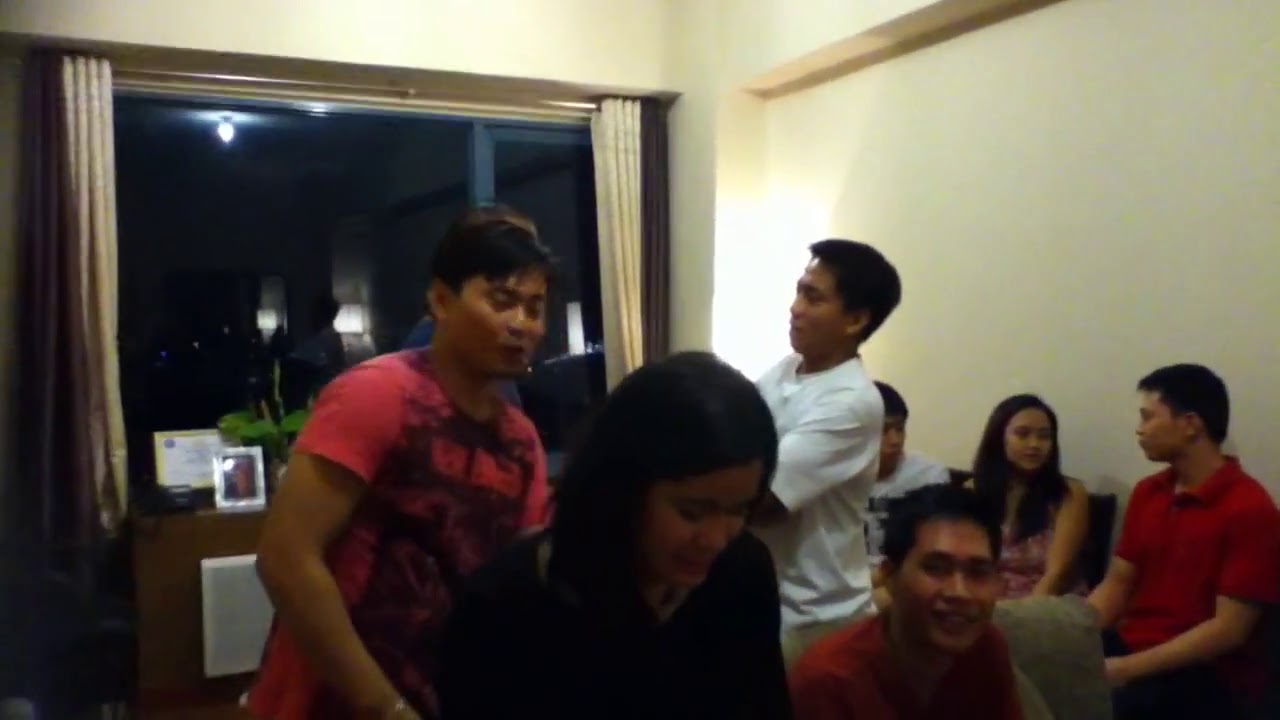In this candid photo, seven individuals of Asian descent are gathered in a small, dimly-lit room with light ivory walls. A large window with tannish curtains dominates the background, reflecting some interior lights, suggesting it is nighttime. The group appears to be casually interacting with each other, with a mixture of standing and seated positions. 

Three people are sitting together on a couch on the right side of the image; a man on the far right, a woman in the middle, and next to her on the left, the half-visible face of another man. In the center of the photo stands a young man with dark hair wearing a white shirt, while seated in front of him is another young Filipino man. Directly in the foreground is a woman with dark hair wearing a dark shirt, looking downward. Behind her, slightly to the left, stands another man with darker skin and wearing a red shirt. Of the entire group, only one person, a woman seated in the foreground, appears to be looking directly at the camera and smiling. There is a hint of a picture and a white square object on a table in front of the window, which adds to the casual, homely atmosphere.